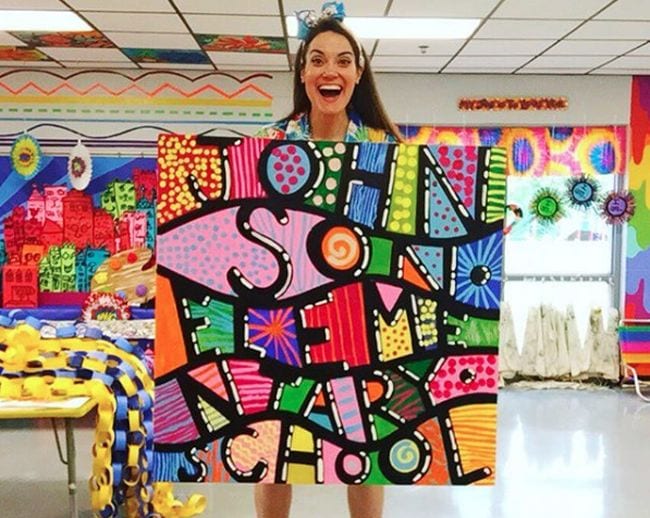In the image, a cheerful teacher with long, straight brown hair adorned with a blue bow smiles widely, showcasing her teeth. She stands in the vibrant, colorful classroom of Johnson Elementary School, holding a whimsical, multicolored sign that reads "Johnson Elementary School" in various shapes and bright hues. Behind her, the room bursts with color, featuring tie-dye curtains, a painted board, and an artist's palette with an array of colors around it. To her right, a desk is covered with a pile of interlinked paper rings. The ceiling displays standard white panels with dark outlines and a horizontal fluorescent light, adding to the distinctive classroom ambiance.